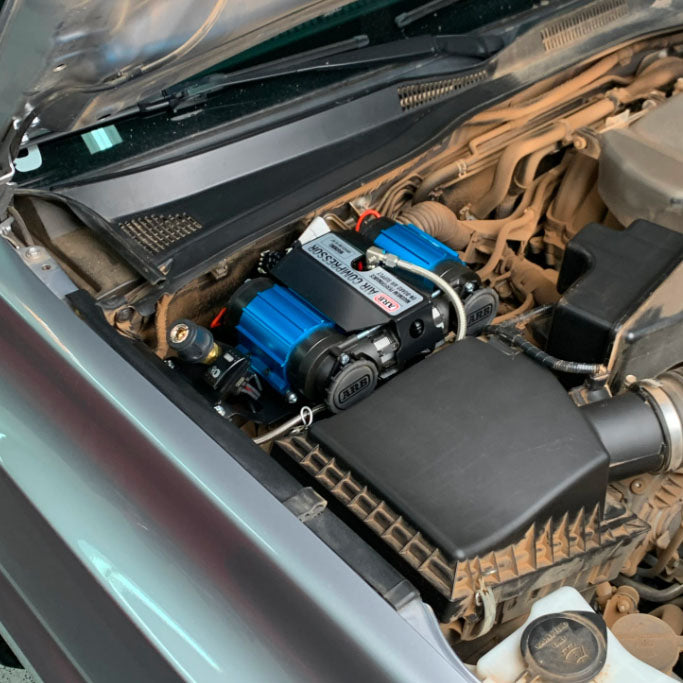This image provides an intricate close-up of the interior of a car engine compartment with the hood open, revealing an array of components. The vehicle appears to be a silvery-gray color. Prominent within the engine bay is a black and blue air compressor, identifiable by a silver label. Visible components include black machinery parts, the oil cap, a carburetor, and several hoses and cables. The cables range in color from beige to sandy brown, suggesting they might be covered in grime. Additionally, the windshield, part of the car's silver exterior, and the windshield wiper fluid cap are seen in the foreground. Overall, the detailed look highlights the utilitarian and somewhat cluttered nature of the engine compartment.